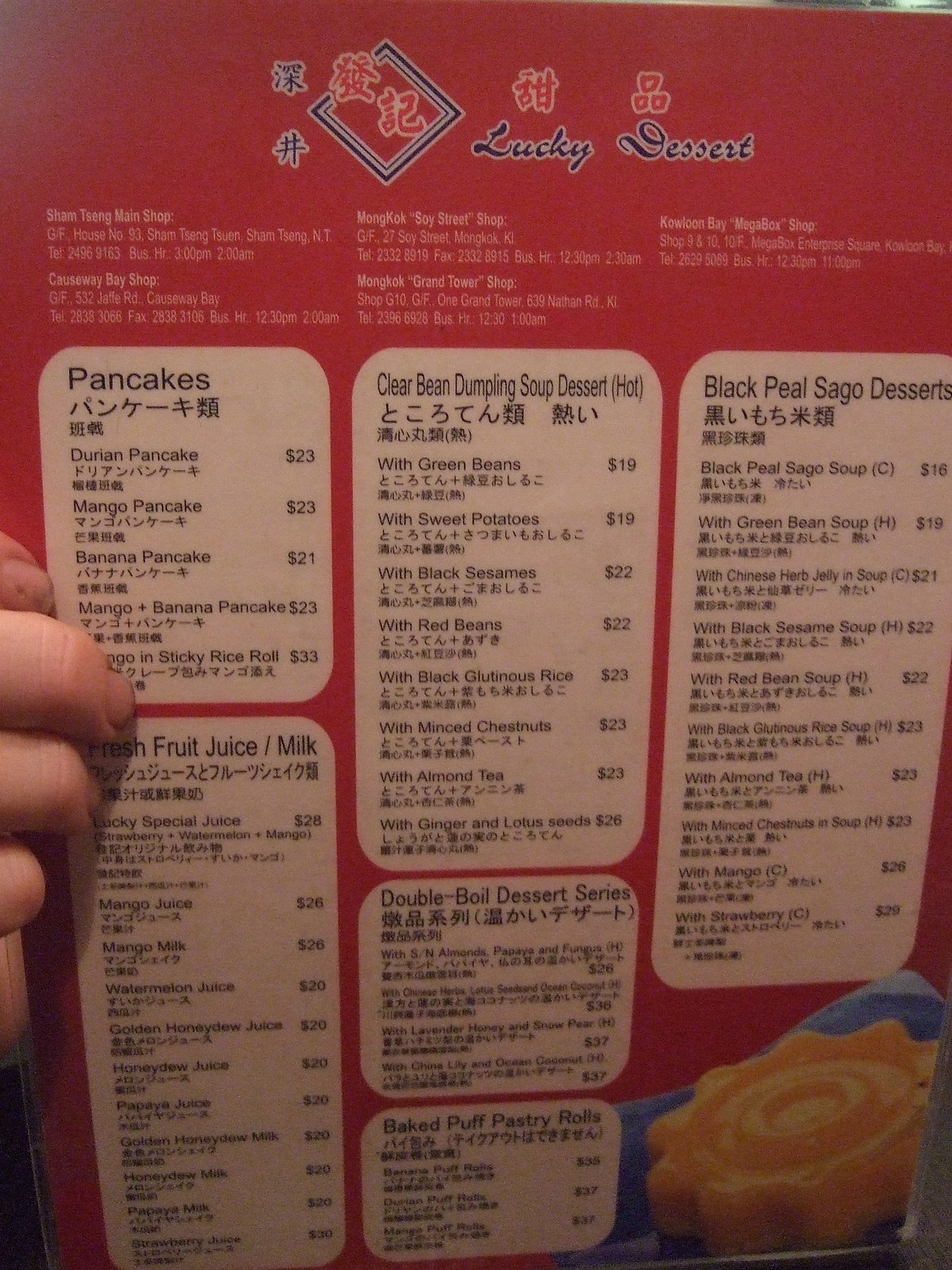This image features a vibrant menu set against a red background in the top right corner, prominently displaying the title "Lucky Dessert". To the left of this title, there is a diamond-shaped emblem adorned with Chinese characters.

The menu is meticulously organized into six distinct sections:

1. **Top Left Section - Pancakes**: This section showcases a variety of flavorful pancakes, including options such as mango, durian, banana, and a combination of mango and banana. Notably, a few fingers are visible holding onto the menu in this section.

2. **Middle Left Section - Fruit Juice and Milk**: Below the pancake section is the fruit juice and milk area, featuring tantalizing choices like mango juice and mango milk.

3. **Top Middle Section - Clear Bean Dumpling Soup Dessert**: Positioned at the top of the middle column, this section announces hot Clear Bean Dumpling Soup Dessert, listing ingredients such as green beans, sweet potatoes, black sesame, and red beans.

4. **Bottom Middle Section - Double Boil Dessert Series**: Directly beneath the soup dessert section, this area introduces the Double Boil Dessert Series, followed by a mention of Baked Puff Pastry.

5. **Top Right Section - Black Pearl Sago Desserts**: In the upper right segment of the menu, there is a selection dedicated to Black Pearl Sago Desserts.

6. **Bottom Right Section - Decorative Plate**: In the bottom right corner of the image, there is a blue plate garnished with a decorative yellow flower, which appears to be crafted from mangoes.

This detailed menu highlights the variety and appealing presentation of the delectable offerings at Lucky Dessert.